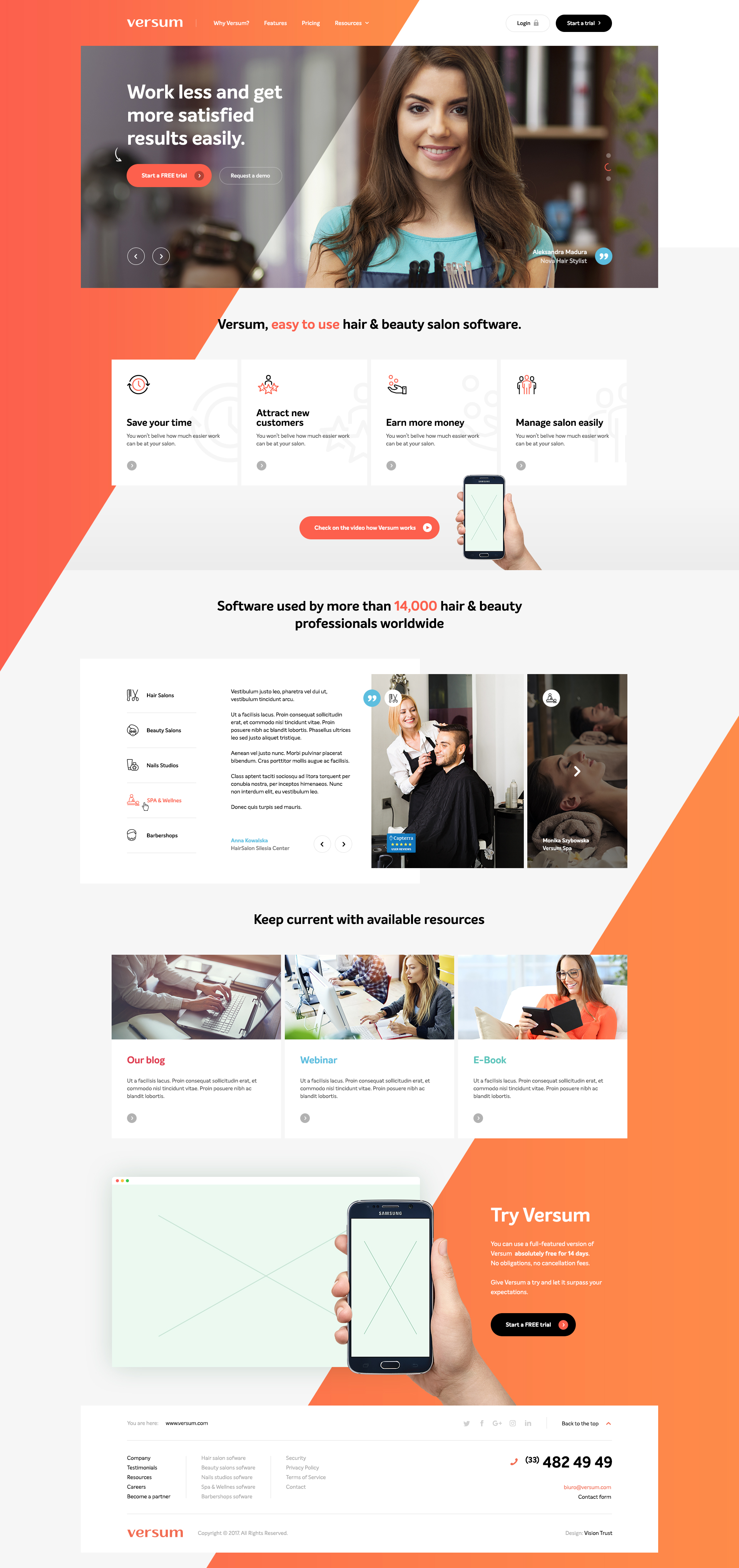**Detailed Caption for Image:**

This image is a comprehensive, vertical screenshot of a webpage from a website or app named "Versum." The top section features the title "Versum" in a distinctive white font located on the top left corner. Adjacent to the title is a menu bar offering various sections: "Why Versum?", "Features", "Pricing", and "Resources," which has a drop-down menu indicated by an arrow. On the far right of the menu bar, there are two prominent buttons—a white one labeled "Login" and a black one labeled "Start a Trial" with a right-facing arrow.

The background of the page is predominantly white, with striking reddish-orange triangular accents in the top left and bottom right corners. Below the menu bar, there is a wide rectangular cover image featuring a brunette woman. Accompanying this image is a subtitle, "Work Less and Get More Satisfied Results Easily," along with options to "Start a Free Trial" or "Request a Demo." In the bottom right of this cover image, the woman is identified as Alexandra Maduro, a Nova hairstylist.

Scrolling down, there is a section titled "Versum: Easy-to-Use Hair and Beauty Salon Software," offering links to four key sections: "Save Your Time," "Attract New Customers," "Earn More Money," and "Manage Salon Easily." Further down, another highlighted section reads, "Software Used by More Than 14,000 Hair and Beauty Professionals Worldwide." This is illustrated by a banner showing a mock-up of the app interface: a menu column on the left and two stock images of people in salons on the right.

Finally, there is a section encouraging users to "Keep Up With Available Resources," featuring three squares with cover images. The bottom of the image showcases a hand holding a smartphone with the option to "Try Versum."